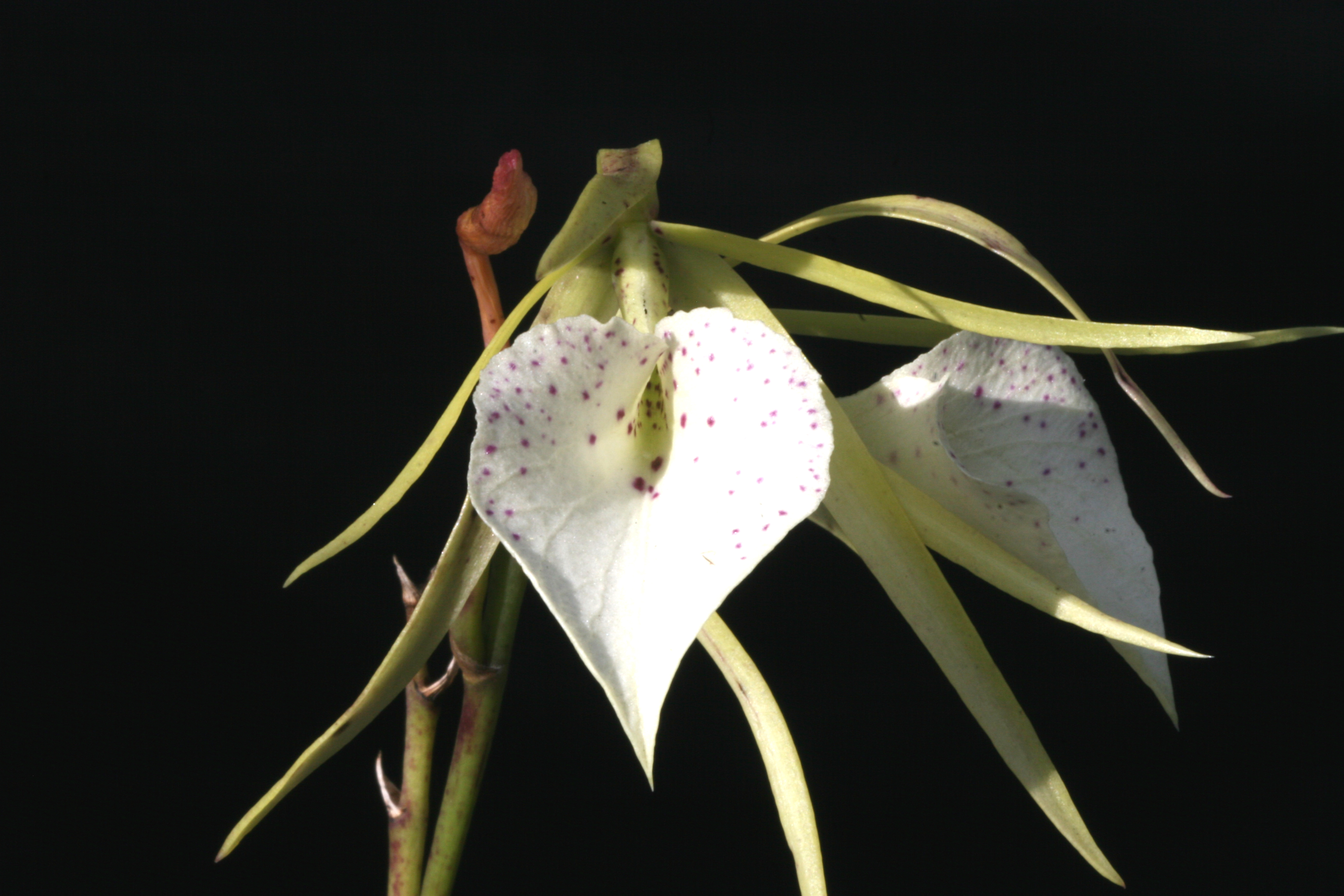This image features a striking close-up of an orchid against a pitch-black background, emphasizing its delicate structure and vibrant colors. The orchid's green stem, with hints of browning, rises from the bottom of the frame, giving way to six or seven light green extensions that droop gently. Two prominent, heart-shaped petals are adorned with pink and purple specks, standing out vividly against the dark backdrop. Behind these petals, a longer red extension capped with a bulbous tip adds an intriguing element to the scene. The juxtaposition of the bright flowers and the stark black background creates a dramatic, almost surreal effect, making the orchid appear as if it is theatrically emerging from the shadows. This visual enigma, with its delicate yet resilient appearance, evokes a sense of both beauty and the mysterious complexity of nature.